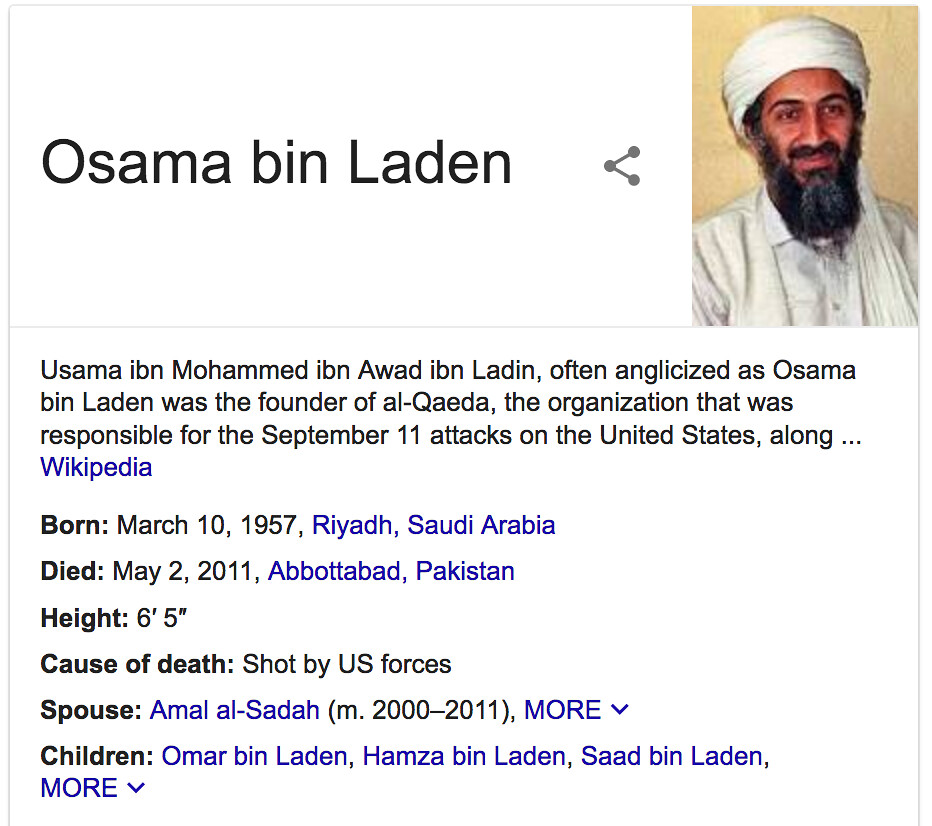This image is a square screenshot of a Wikipedia page, primarily white with some text highlighted in blue. In the top right corner of the page, there is a photograph of Osama bin Laden. He is depicted with brown skin, a long brown beard, and wearing a white headdress and robe. To the left of the photograph, the text "Osama Bin Laden" is prominently displayed in black font. Below this, more detailed biographical information is provided: "Osama Ibn Muhammad Ibn Awad Ibn Laden, often anglicized as Osama Bin Laden, was the founder of Al-Qaeda, the organization that was responsible for the September 11th attacks on the United States." Additional information includes his birth date (March 10, 1957) in Riyadh, Saudi Arabia, and his death date (May 2, 2011) in Abbottabad, Pakistan, noting that he was shot by U.S. forces. Other details such as his height (6 feet 5 inches), and family information including his spouse Amal al-Sadah (married from 2000-2011), and children Omar bin Laden, Hamza bin Laden, and Saad bin Laden are also listed. The content and structure of the text are organized from top to bottom, left to right, and the page typography is mostly in black with some entries in blue, signifying links.